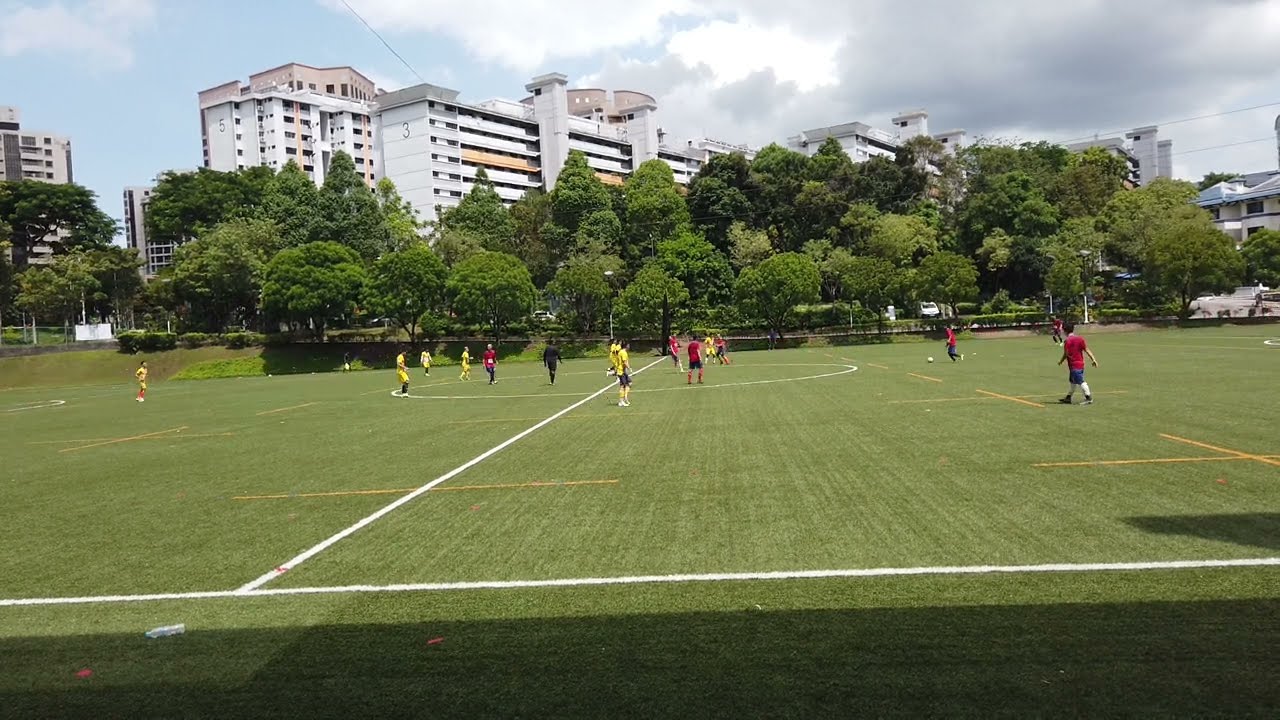This vibrant outdoor photograph captures a lively soccer game unfolding on a lush, green field under a dynamic sky. The soccer field, detailed with crisp white boundary lines and prominent goal posts, dominates the foreground. While the teams, clad in yellow and red jerseys paired with black shorts, play in the center, a referee in an all-black outfit oversees the match. Though the players appear small and indistinct, possibly indicating a youth game, their dynamic energy is palpable.

The foreground is partly shaded, likely by a building or stadium stands. Beyond the field, a dense row of trees, boasting heavy canopies of verdant summer foliage, forms a natural boundary. Nestled behind the trees, a substantial white building stands tall, potentially serving as an apartment complex or hotel. Its main structure features a flat roof, while an adjacent section to the left sports a distinctive red peaked roof. The scene is capped by a captivating sky, with white puffy clouds giving way to darker, stormy hues in the upper right corner, adding dramatic contrast to the otherwise bright daytime setting.